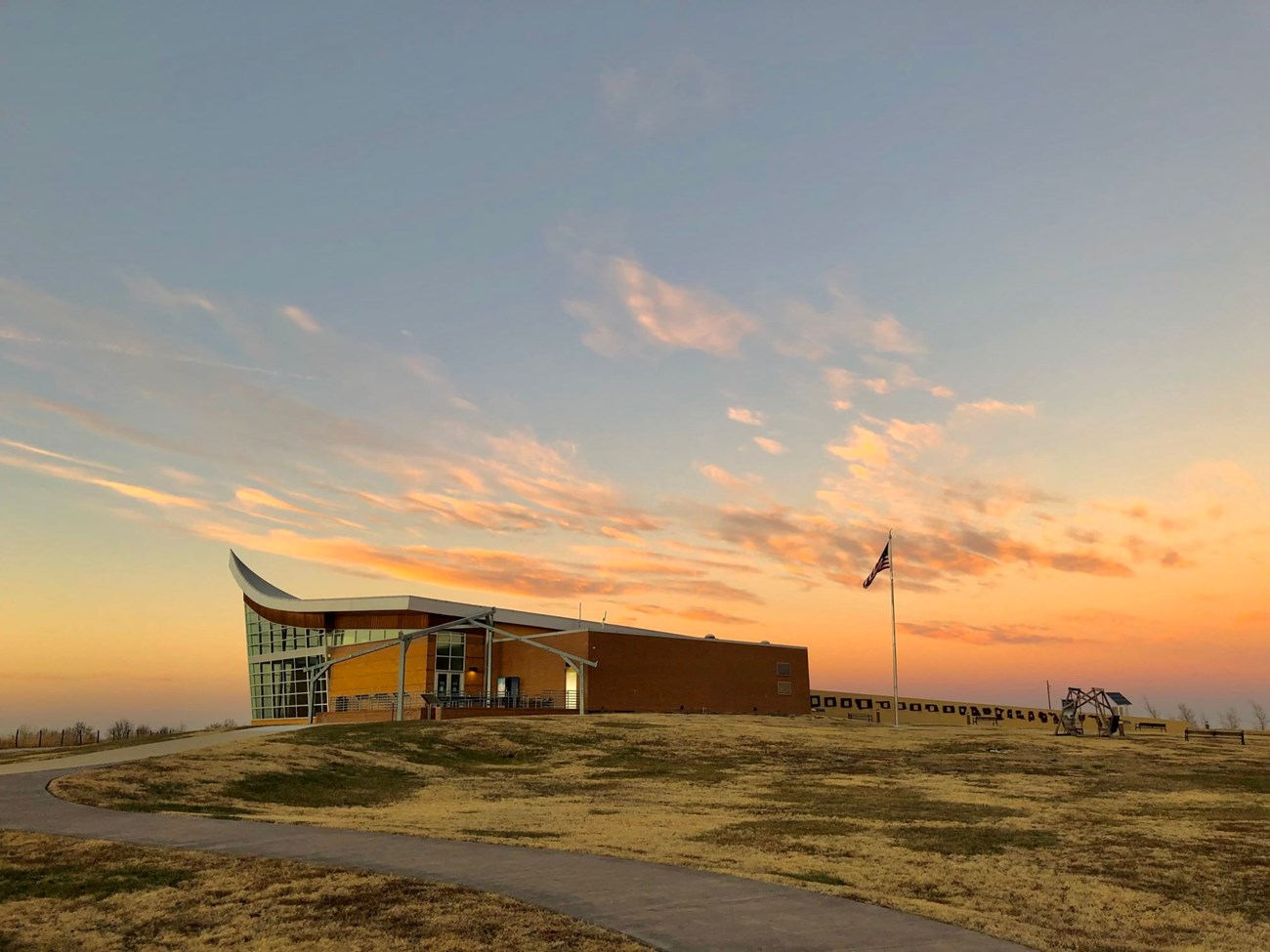The photograph captures a strikingly modern yet somewhat vintage-looking building, possibly from the 1950s or 1960s, situated on a hilltop. The unique architectural design features a sloping roof that resembles an ocean wave, ascending into a partly glass façade on the left side. This side of the building is accentuated by metallic pieces that frame a patio area, possibly with a couple of chairs visible. The structure is primarily composed of brick, with a combination of yellow and goldish-tan hues.

In front of the building, a concrete pathway and a small paved road lead up towards the entrance. This entryway is further complemented by a large flagpole displaying an American flag, reinforcing the possibility that this is an institutional building like a school or office. Extending out from the main building is a long, narrow section adorned with numerous small brown windows.

The photograph likely captures either sunrise or sunset, as suggested by the orange-tinged clouds against a blue sky. The surrounding landscape appears somewhat isolated, with dormant light brown grass scattered with some splashes of green. Bare-branched trees are visible in the background, enhancing the tranquil yet somewhat deserted atmosphere of the scene.